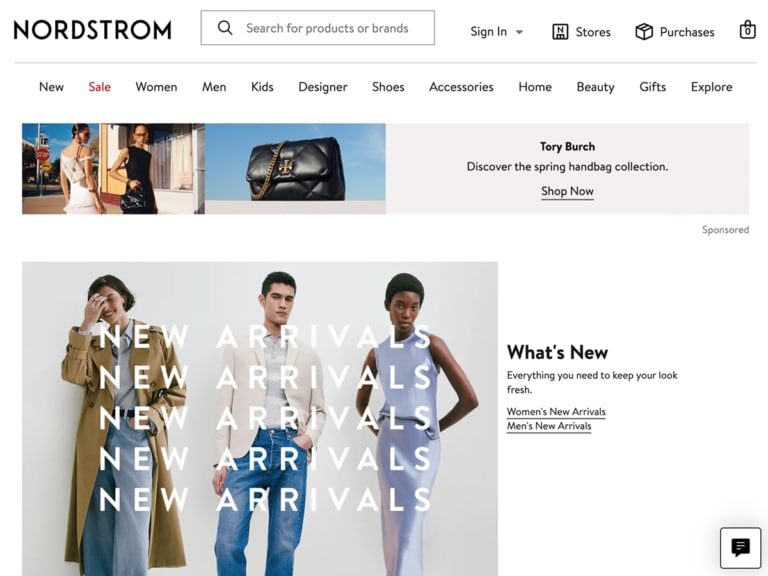The screenshot depicts a web page from Nordstrom, showcasing various navigational elements and advertisements prominently. 

At the top left corner, the Nordstrom logo is displayed in black, consistent with their usual branding. Adjacent to the logo, there is a search box designed for easy access. Following this on the same top row are several icons: a sign-in button, a store locator, a 'purchases' section, and a shopping cart icon, which currently shows zero items.

Beneath the top row, another set of navigational buttons is present, likely representing different departments within the Nordstrom website. These buttons, smaller than those above, include categories like New, Sale, Women, Men, Kids, Designer, Shoes, Accessories, Home, Beauty, Gifts, and Explore. Notably, the 'Sale' button is highlighted in red, possibly indicating it has been selected.

Below these navigation options, there is a small advertisement featuring two adjacent photos. The right-hand side showcases a Tory Burch black bag with the tagline "Discover the Spring Handbag Collection," while the left-hand side presents a smaller image of two women. 

Directly underneath this ad, a larger image spans the width of the section, highlighting three models dressed in different outfits. Overlaid text in white reads "New Arrivals" repeatedly down the center of the image, likely drawing attention to the latest fashion introductions. The accompanying text further elaborates on the new items available.

Overall, the webpage highlights navigational ease with clear categorization and visually engaging advertisements to draw user attention to specific promotions and new collections.